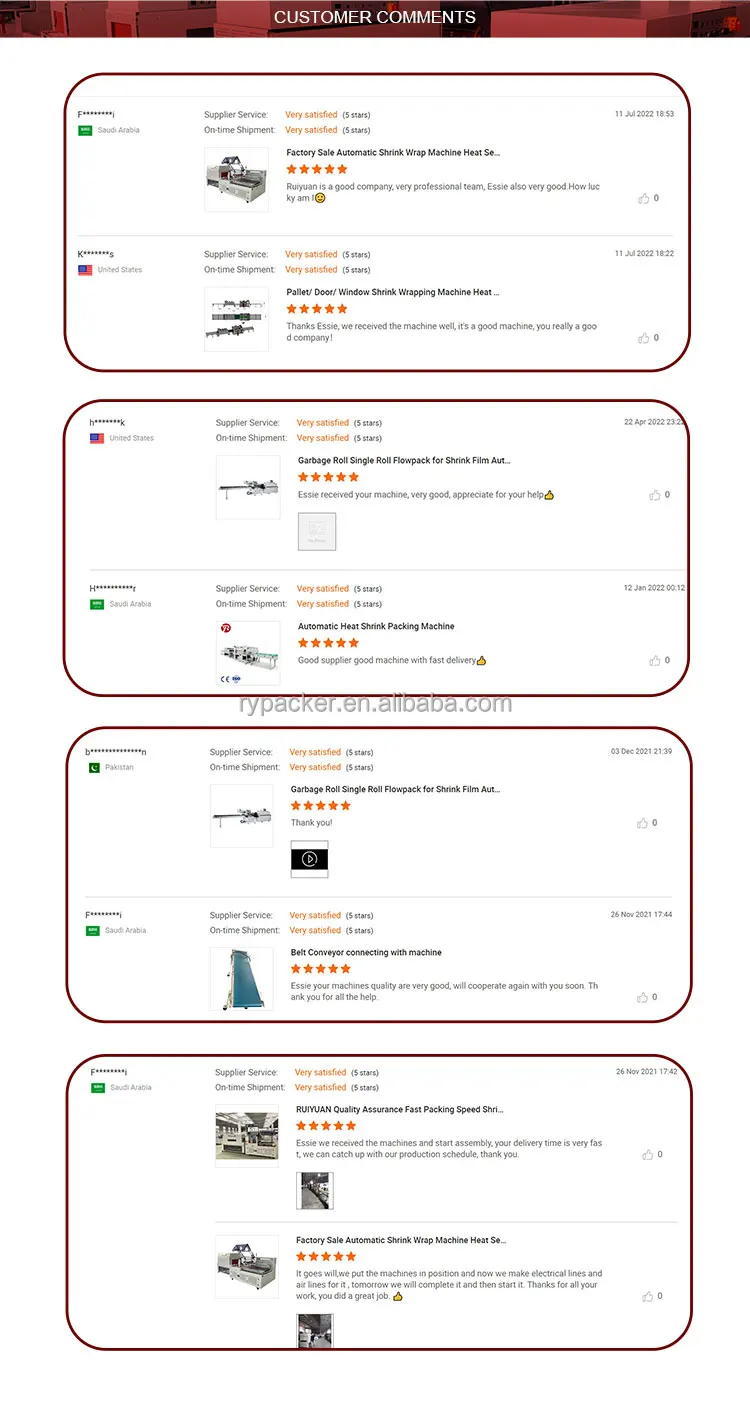This image, sourced from a website, features a heavily blurred visual with an identifiable section titled "Customer Comments" in white letters set against a black and white background at the top. Below this header, a series of rectangular sections, all outlined in black, are aligned vertically. Each rectangle contains images of two objects accompanied by a five-star rating. Beside these images, there are comments or additional information, though the details are too blurry to discern. This consistent layout of dual objects, five-star ratings, and corresponding text continues throughout the rectangles, catering to a uniform presentation style.